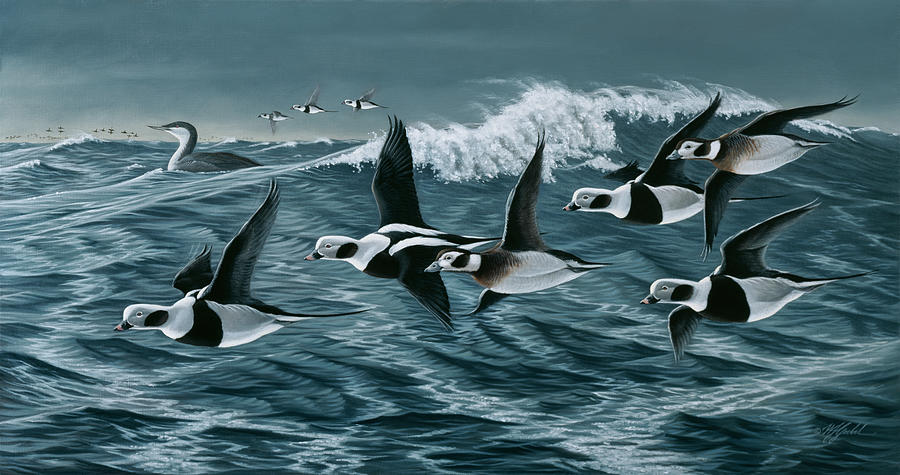This image is a painting of birds flying over a stormy, dark blue ocean with white-capped waves. The scene features several seabirds with distinctive black and white coloring, orangey-red beaks, and black wings. Six birds fly in a close formation in the foreground, appearing sharp and in focus, while another bird floats on the water's surface. Additional birds can be seen, blurred, in the stormy, gray sky background. There is cursive writing in the bottom right-hand corner of the painting, though it's too distant to read. The overall mood is dramatic, capturing the turbulent nature of the ocean and the determined flight of the seabirds through the storm.